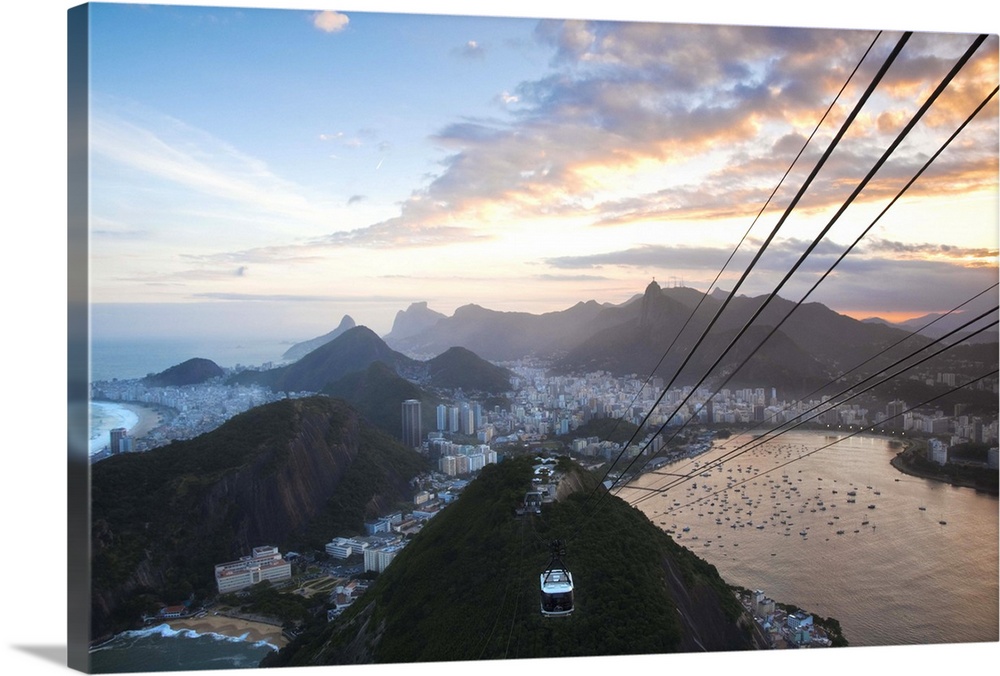This color photograph captures a scenic aerial tramway suspended on cables, gracefully traversing between towering, tree-covered peaks above a sprawling cityscape. The tramway car, metallic silver with black-tinted windows, is seen emerging towards the camera, its cables extending from the upper right of the image towards a distant mountain. The mountainous landscape is rich with greenery, resembling the foothills of a larger mountain range. To the right, a vast bay brimming with moored boats blends seamlessly into the city beyond, characterized by an array of structures from towering skyscrapers to modest buildings. Beyond the city, jagged peaks rise majestically, encircling the scene. To the left, the expanse transitions to open ocean, with a visible beach and clusters of smaller buildings. The sky is a picturesque blend of blue and cloud, with the time of day marked by the sun either rising or setting, casting a beautiful array of oranges, yellows, and pinks onto the horizon, reflected softly in the scattered clouds.